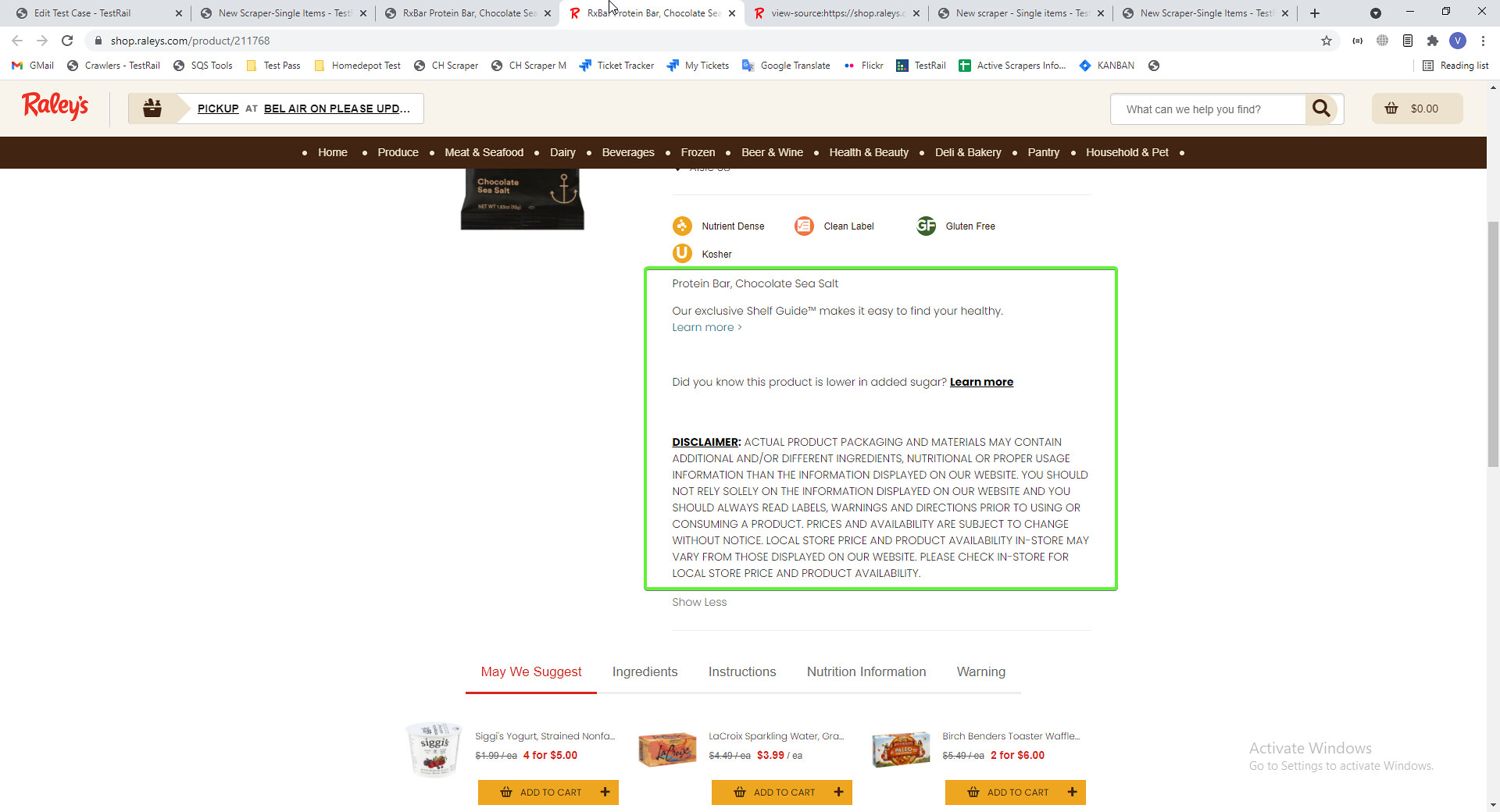A screenshot of a desktop computer displaying the Chrome web browser on the Raley's grocery store website. The user has scrolled slightly down from the top of the page, centering the focus on a prominent neon green box containing informative text. The text within the box highlights a product: "Protein bar, Chocolate Sea Salt." It mentions Raley's exclusive shelf guide, designed to help customers easily identify healthy options, with a prompt to "Learn more." Additionally, it notes that this particular product is lower in added sugar and offers another "Learn more" link. Below this, there is a disclaimer stating that packaging differences may occur, along with a reminder to check nutrition labels and a note that prices are subject to change.